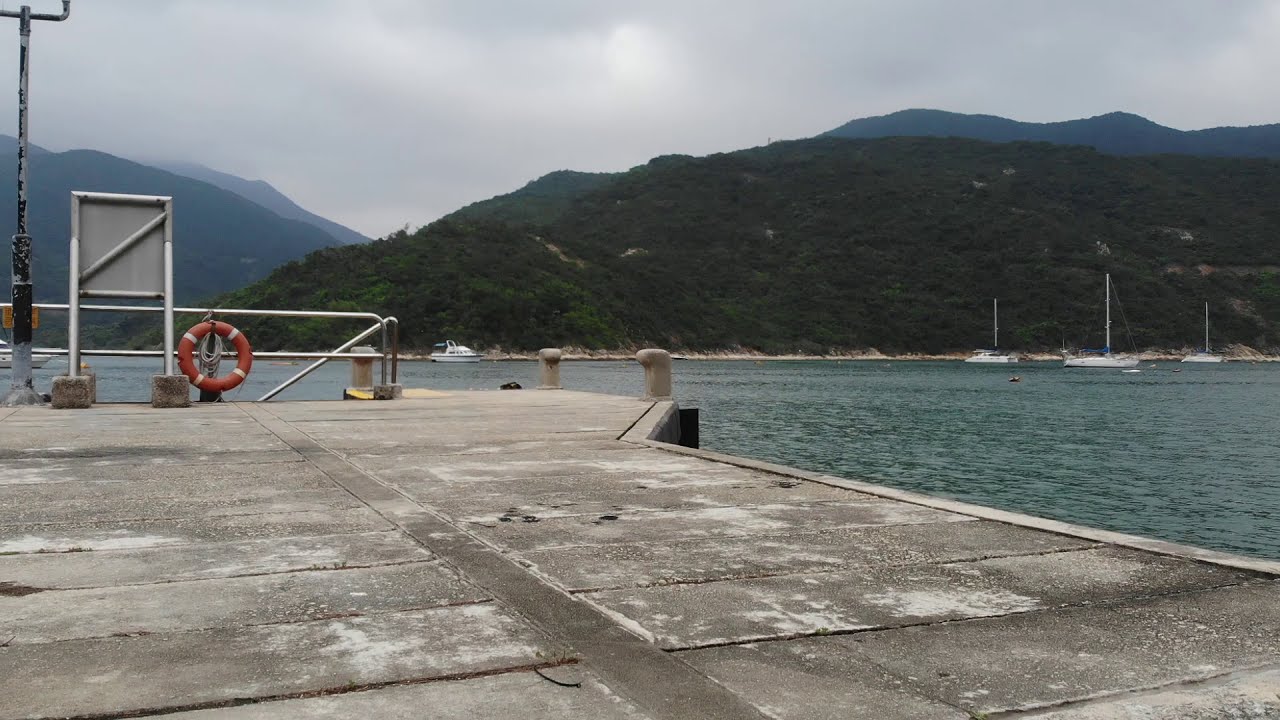The photograph captures a concrete pier extending out onto calm, greenish-blue water. The dock itself shows patches of dark gray or brown, with some areas seemingly affected by black mold. On the right side, a silver railing includes a distinctive orange-red life-saving ring, marked with four white stripes. This ring is securely fastened to the railing. The scene is set under an overcast sky, with clouds hanging low over the towering, green mountains that frame the background. These mountains are lush with forest and shrubs, giving a sense of dense greenery despite the cloudy weather. Several sailboats, with their masts upright but sails down, are scattered across the bay, enhancing the tranquil atmosphere. A staircase descends from the pier, suggesting a route to board boats. The overall scene, taken in what appears to be summertime, evokes a serene yet somber mood due to the overcast conditions.